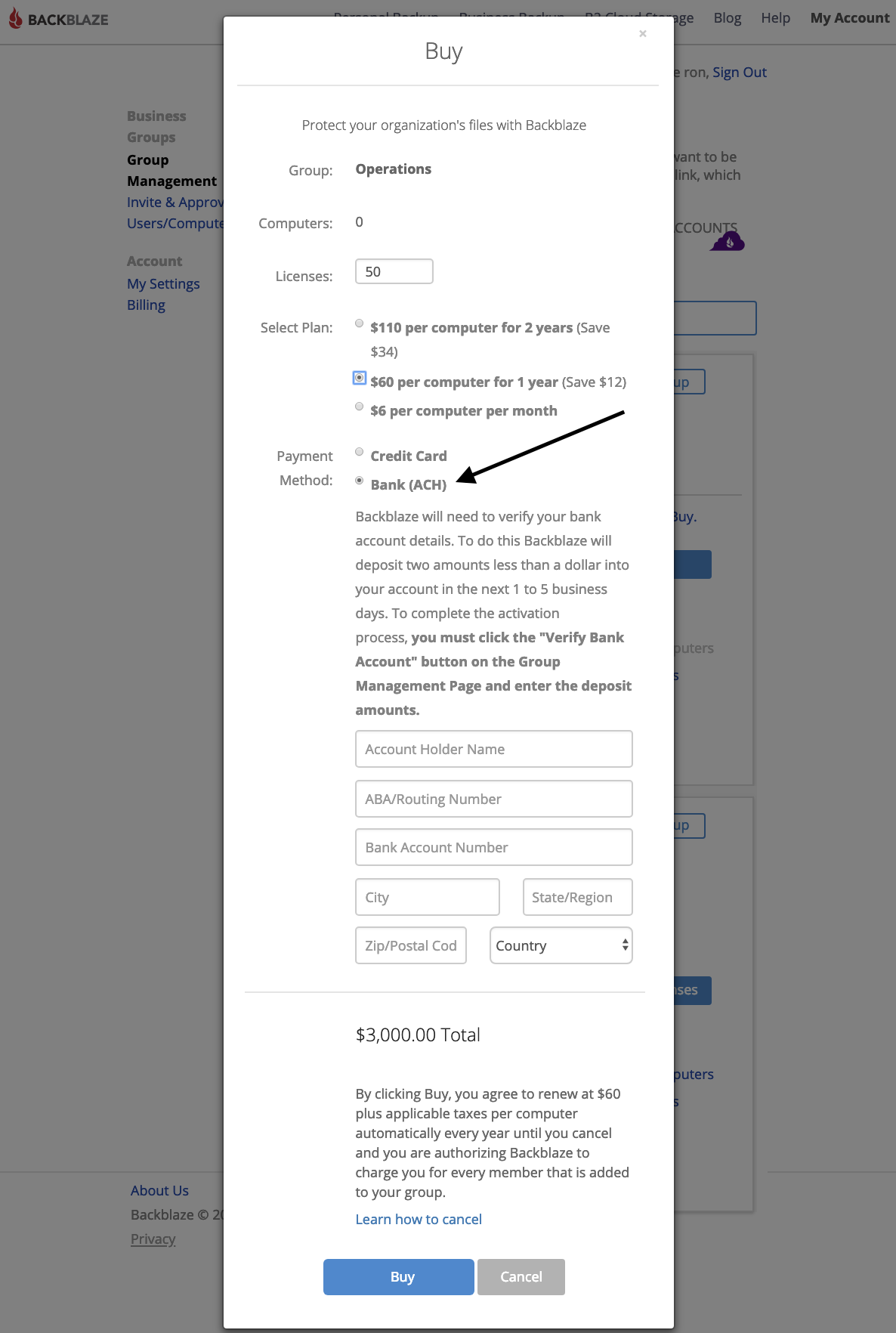This vertical rectangular image prominently features a centered, crisp white overlay on top of a blurred background. At the top of this overlay, the word "BUY" is displayed in bold black font. Below this, a horizontal line separates the header from the text. The text reads, "Protect your organization's files with," followed by some smaller, less legible text. Further down, the bolded phrase "Group with Operations" is visible, with details listed vertically below it: "Computers: 0" and "License: 50" (in a small rectangular box).

Next, a section labeled "Select Plan" features three bullet points for different plan options. The middle option is highlighted with a turquoise border, stating "$60 per computer for one year" and "Save $12" in parentheses. Under this section, a black arrow points downward to a section titled "Payment Methods," detailing two bullet options: "Credit Card" and "Bank (ACH)." The arrow points toward the ACH option.

Small text explains that Backblaze will deposit two amounts under a dollar into the provided bank account within one to five business days. Users must click "Verify Bank Account" on the group management page and enter the deposited amounts to complete activation.

At the image's bottom, two horizontal buttons are present. The larger button reads "BUY" in white font on a blue background, while the smaller, light gray button reads "CANCEL" in white font. Between the text sections and buttons, fields for name and address information can be filled. Additionally, a section indicating "$3,000 Total" and a waiver stating, "By clicking buy, you agree to," can faintly be made out.

The backdrop of the image bears the Backblaze logo in the upper left corner, featuring a red icon and the word "BACKBLAZE" in all capital letters. Along the left side of the white overlay, non-overlay text reads "Business," followed by "Groups," "Group Management," and another slightly illegible word.